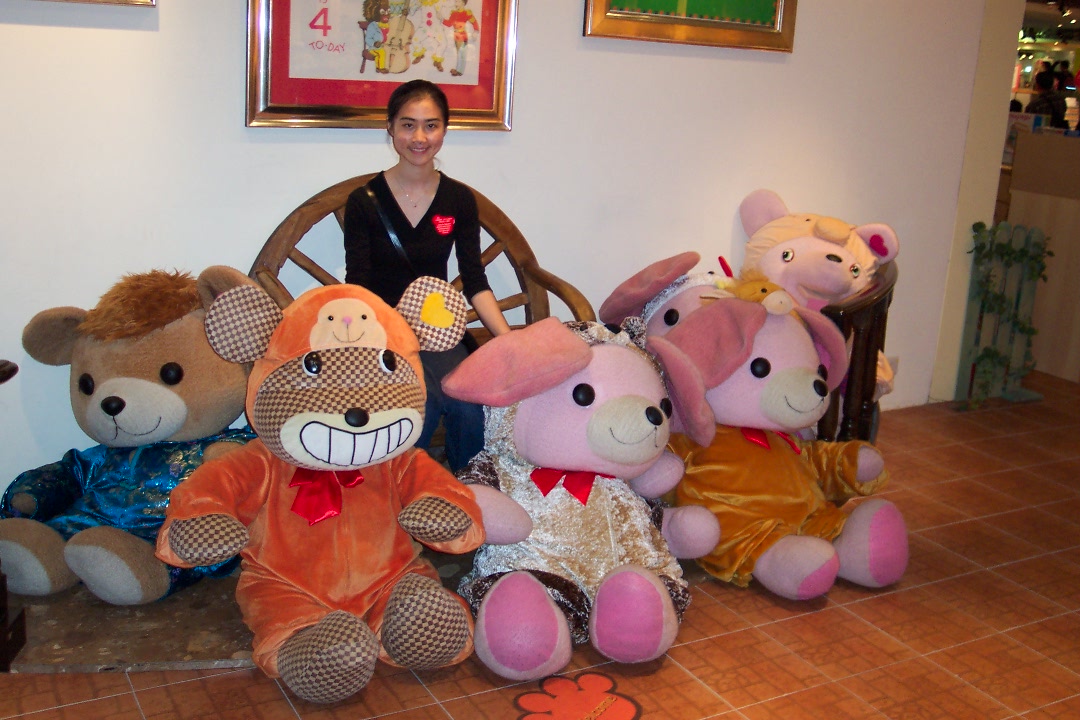In this indoor color photograph, a young Asian woman, who appears to be in her early twenties, is seated on a brown wooden bench against a white wall. The woman, dressed in a black dress, smiles warmly at the camera from behind a playful assortment of oversized stuffed animals, each at least a meter and a half tall. Arranged in a semicircle in front of her are these giant plush toys: to her left is a traditional teddy bear donning a blue outfit, while in the center, another teddy bear sports an orange jacket and hat, distinguished by a checkered pattern on its brown body. To the right, there is a pink animal resembling either a dog or a pig, accompanied by two other similar pink creatures with long ears, pink feet, legs, and faces. The scene is set in what appears to be an educational environment, possibly a daycare or kindergarten, suggested by the childlike illustrations on the walls and the framed picture behind her. The floor features a brown checkered linoleum pattern, adding to the whimsical atmosphere of the setting.